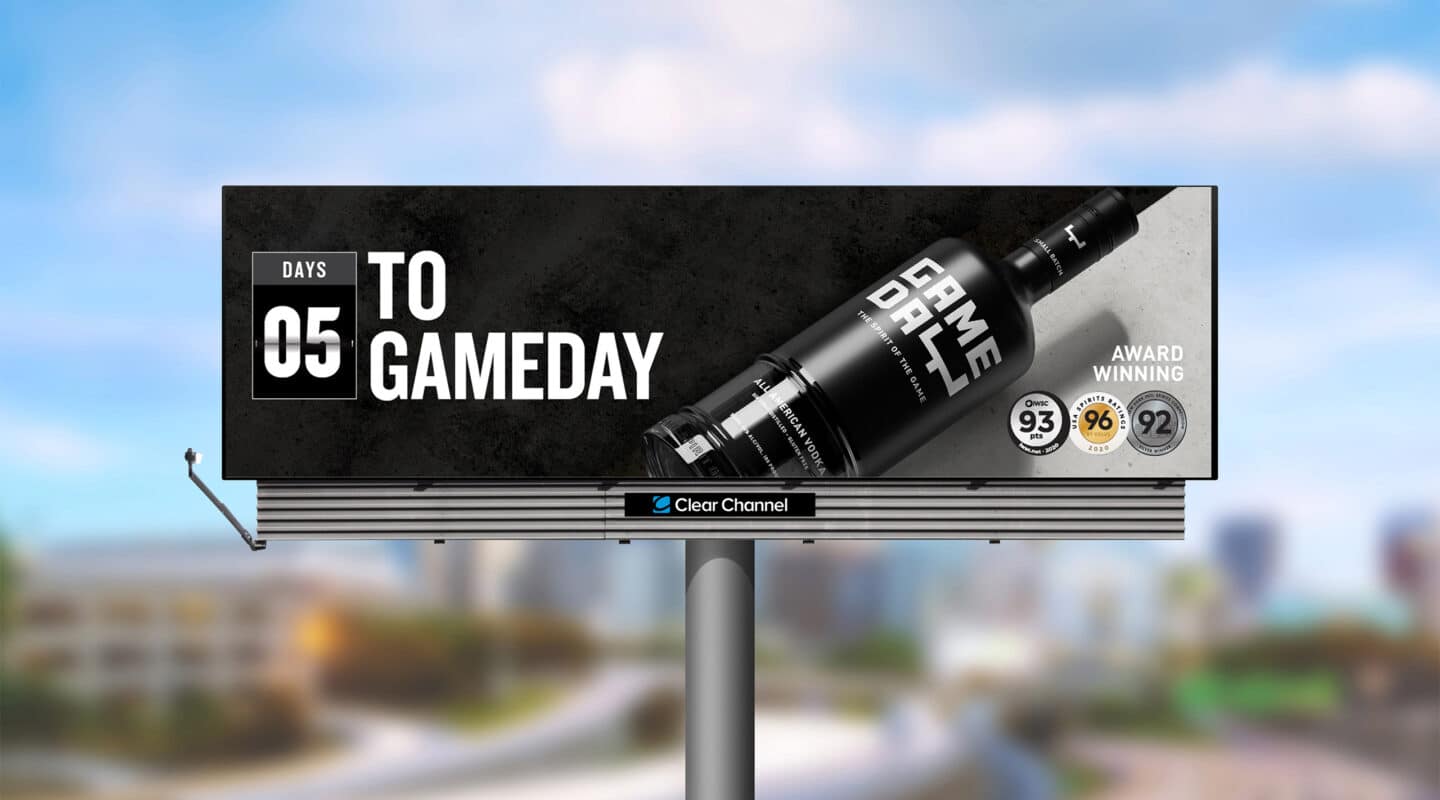This color photograph features a billboard prominently displayed against a blurred background. The billboard, a long rectangle mounted on a sturdy metal pole, showcases a predominantly black design with a diagonal gray patch on the far right side. Central to the advertisement, it reads, "Days 05 to Game Day," with emphasis on a sleek black liquor bottle, positioned on its side, labeled "Game Day." Intriguingly, the 'Y' in "Game Day" is creatively shaped like a football goal post. The tagline, “The spirit of the game, All-American Vodka,” underscores the brand's sporty theme. Notably, the bottle casts a distinct shadow onto the gray section of the billboard. In the bottom right corner, the billboard proudly declares "Award Winning," accompanied by three circles boasting ratings of 93, 96, and 92, though the finer details in these circles remain indistinct. At the very bottom, the name "Clear Channel" denotes the advertising company.